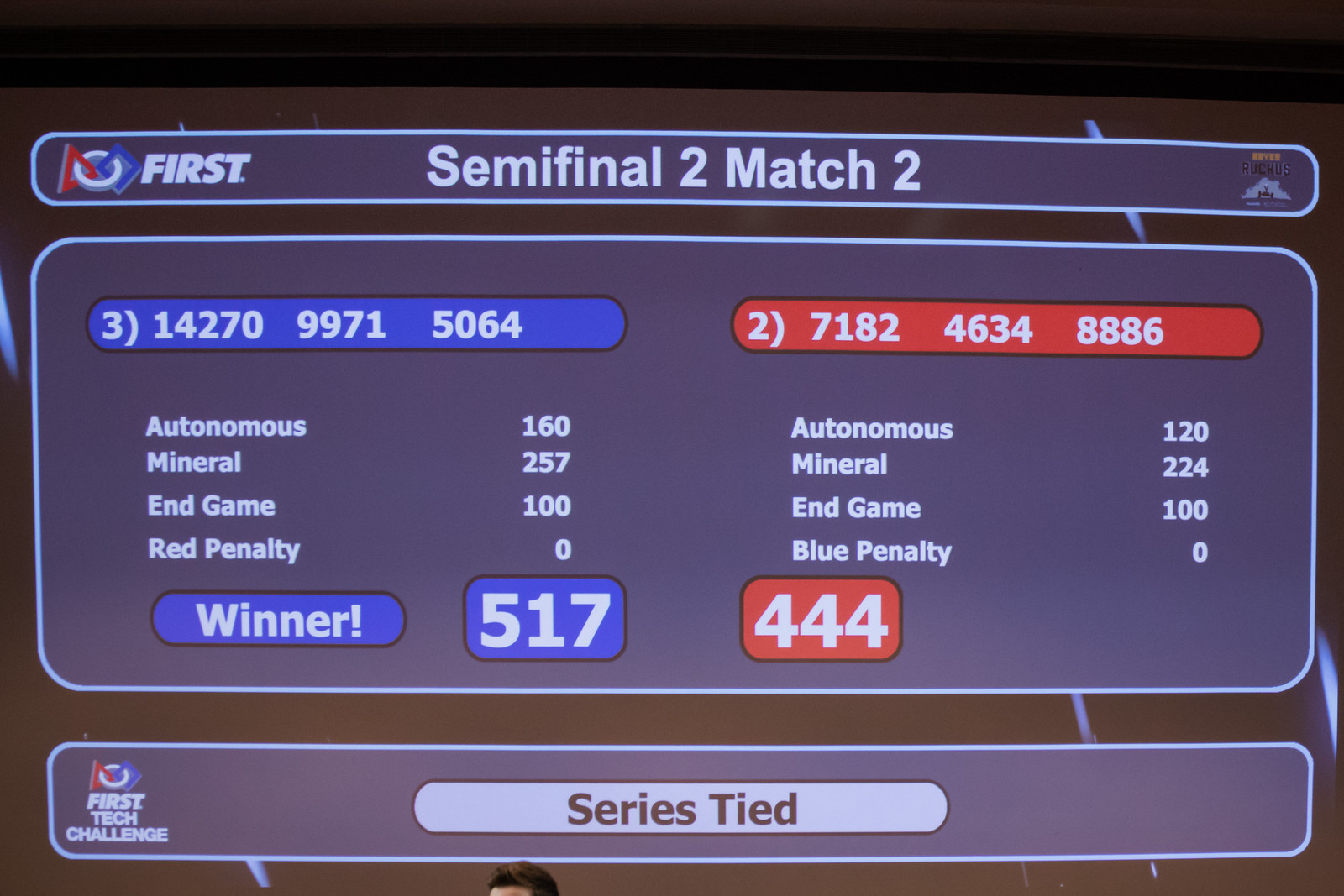The image depicts a close-up of a large projected scoreboard, likely from a competition. Dominating the screen is an interlocked triangle, square, and circle logo at the top left corner, with the text "First Tech Challenge, Semi-Final 2, Match 2." Below, the scoreboard details the scores for both teams. The blue team, labeled as "number three," scored 517 points, winning against the red team, labeled as "number two," which scored 444 points. Categories dividing the score include "Autonomous," "Mineral," and "End Game." The red team has a "Red Penalty" section, while the blue team has a "Blue Penalty" section. The blue team is declared the winner, and at the bottom of the screen, it notes that "the series is tied." The scoreboard is prominently colored in black, gray, blue, red, white, off blue, gray, and tan. A person’s head is visible at the bottom, further indicating it is projected onto a large screen, taking up most of the image's view.